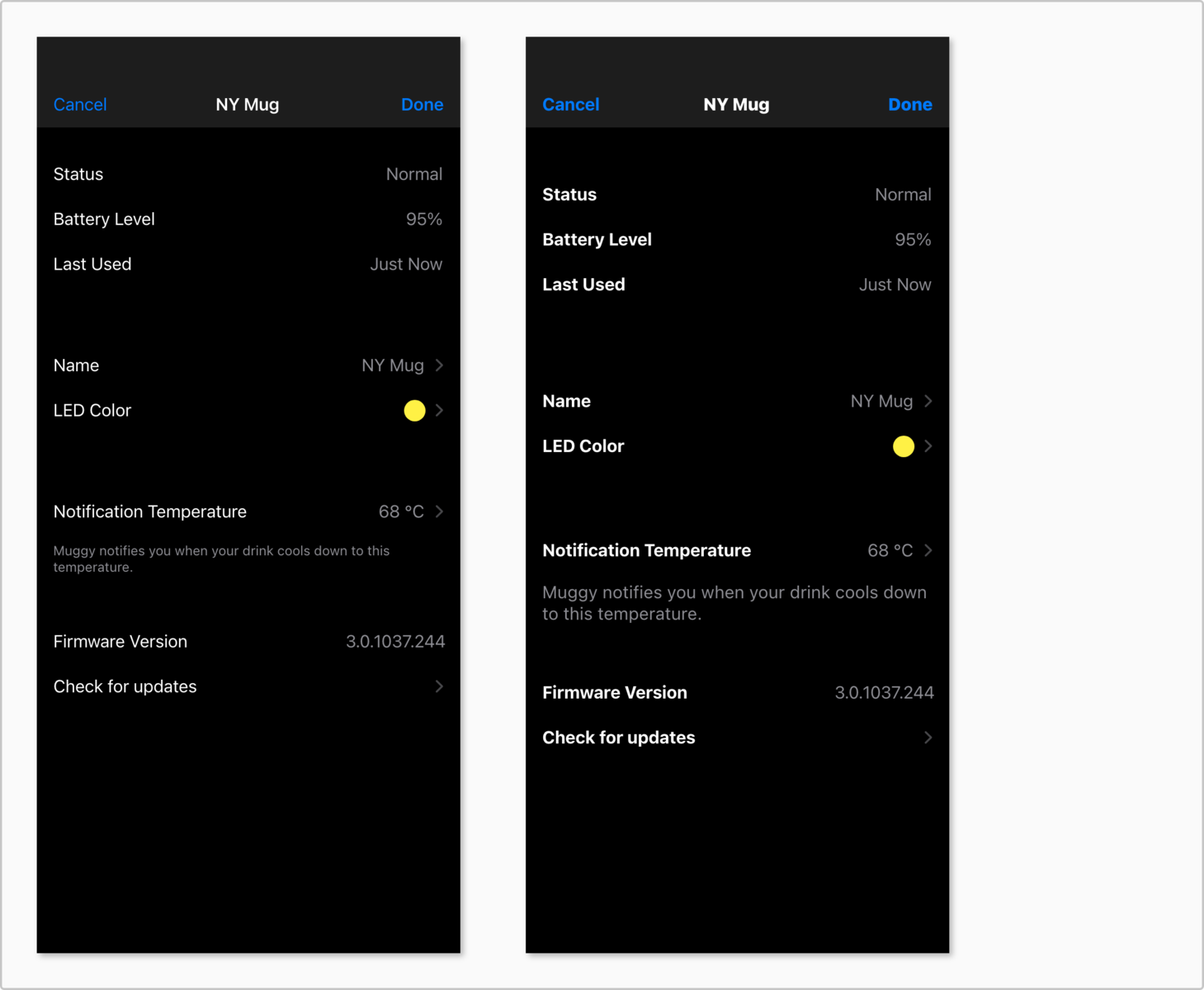The image consists of two side-by-side screenshots from a cell phone display, each showcasing the status of a smart mug. Both screenshots feature a blue navigation bar at the top, with a "Cancel" link on the left, "NY Mug" centered in white, and a "Done" link on the right.

The left screenshot provides a detailed status of the mug:
- **Status**: Normal
- **Battery Level**: 95%
- **Last Used**: Just now
- **Name**: New York Mug
- **LED Color**: Yellow
- **Notification Temperature**: 68°C (indicated as "muggy hotlines" which is a typo; should be "mug notifies")
- Notifies when the drink cools to this temperature
- **Firmware Version**: 3.0.1037.244
- Option to **Check for Updates**

The right screenshot shows identical information, but with slight differences:
- The text appears slightly brighter and larger compared to the left screenshot.

Both screenshots have a black background with white text, except for the blue hyperlinks at the top. While the white text on the left screenshot is standard, the right screenshot features text that is distinctly brighter and more prominent.